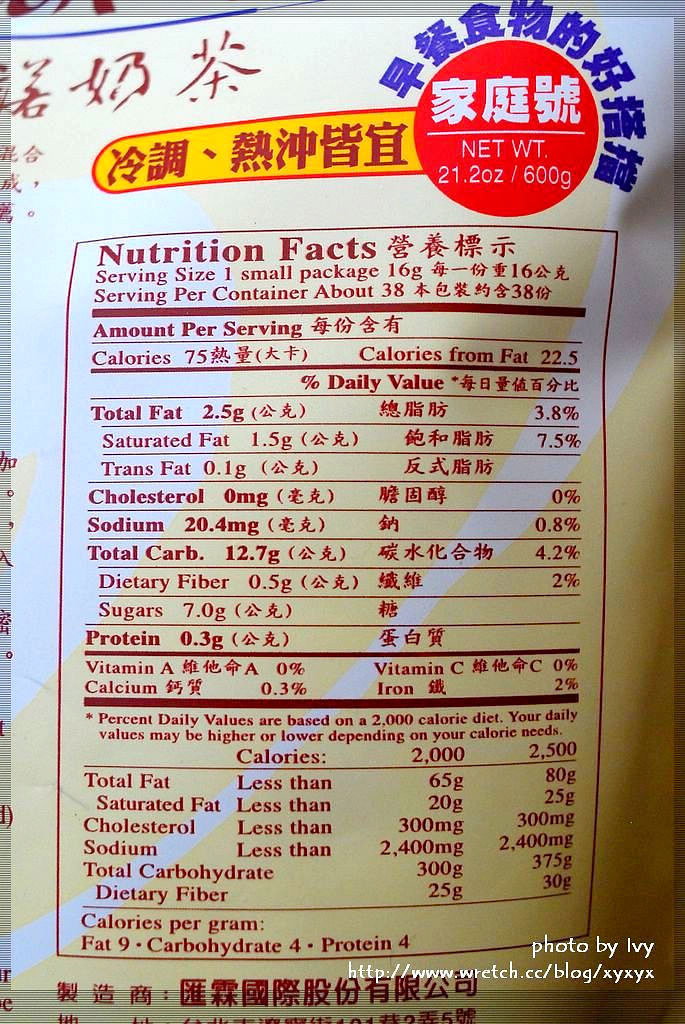The image depicts the back of a food package, prominently featuring a nutrition facts label primarily in Chinese, though key sections and titles are in English. The package is white, with the nutrition text in red. At the top of the label, there is a red font on a yellow background, adjacent to a red circular area with white text, encircled by blue text. The nutritional information details a serving size of one small package (16 grams) with about 38 servings per container. Each serving contains 75 calories, 22.5 from fat, 2.5 grams of fat, 1.5 grams of saturated fat, 0.1 grams of trans fat, 0 grams of cholesterol, 20.4 milligrams of salt, 12.7 grams of carbs, 0.5 grams of dietary fiber, 7 grams of sugar, 0.3 grams of protein, 0% Vitamin A, 0.3% calcium, 0% Vitamin C, and 2% iron. Additional information is provided below these details. A note in the lower right-hand corner credits Ivy with the photo, along with a URL: http://www.wretch.cc/blog/xyxyx.